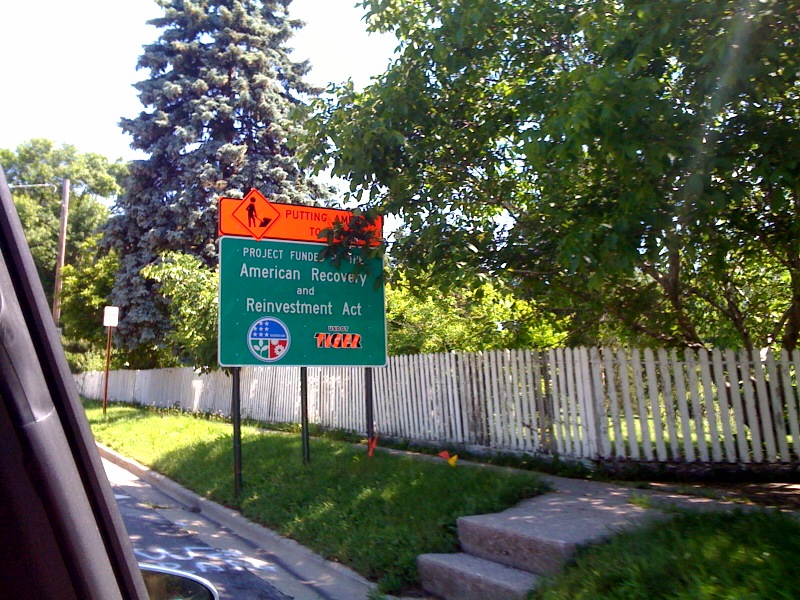In this photograph taken from within a silver car, the view from the passenger side window frames a scene of suburban tranquility. The side view mirror and part of the car's middle frame are visible in the foreground, anchoring the perspective. Beyond the vehicle, an expansive swath of vibrant green grass stretches out between the curb and a picturesque white picket fence. A street sign, supported by three metallic poles, commands attention. At the top, a bright orange rectangular sign boldly displays the word "PUDDING," though the remainder of the text is obscured by a tree branch. Below it, a green sign with a white border reads, "Project funded by American Recovery and Reinvestment Act." The entire sign is lightly shaded by the leaves of a tree situated just beyond the fence. In the serene scene, two stone steps lead from the street, invitingly climbing up to the picket fence and completing the idyllic suburban setting.